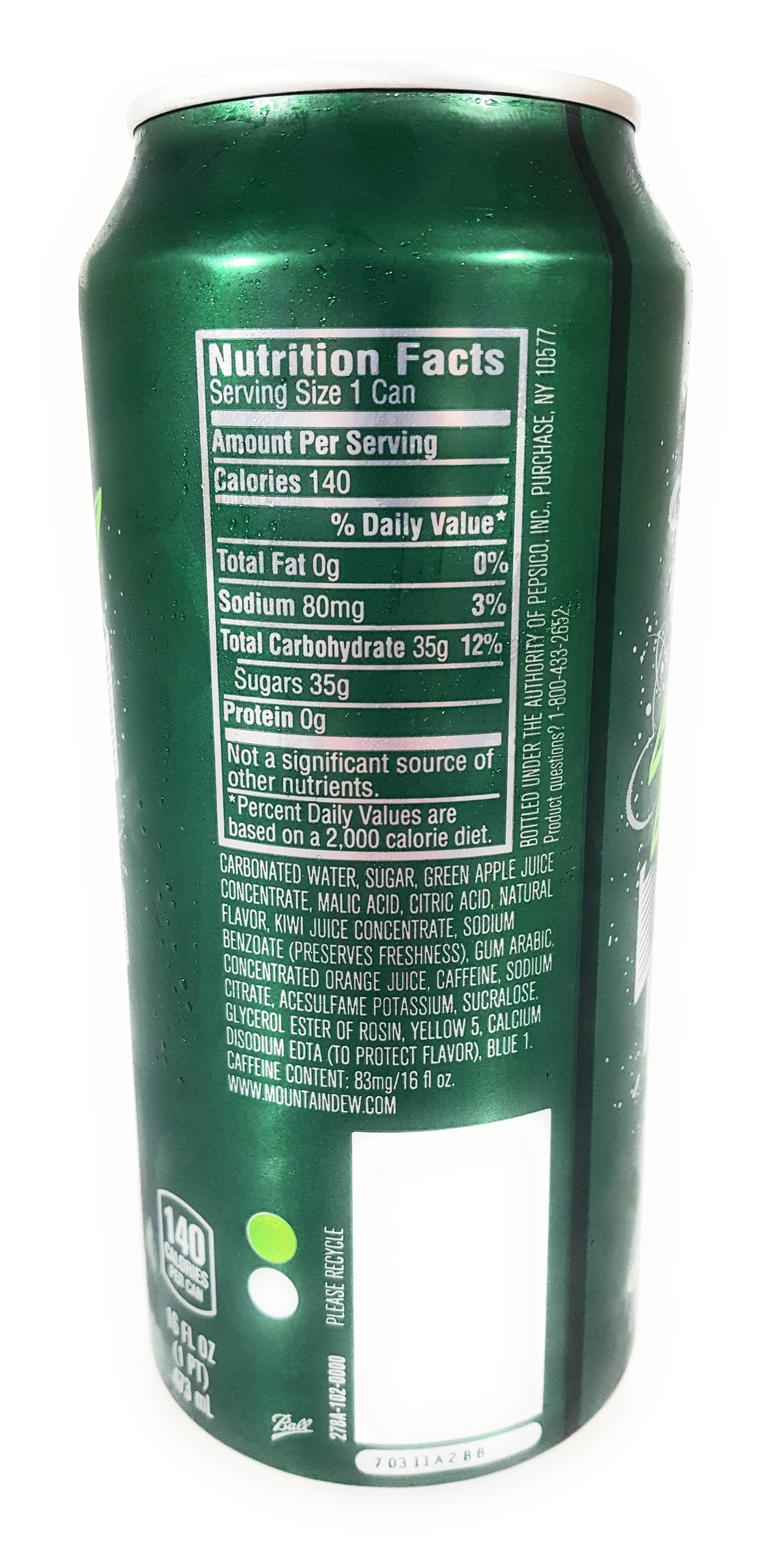This image features a tall, jade-green aluminum can, predominantly showcasing the nutritional facts label on its side. The can, possibly a variant of Mountain Dew or a similar soft drink, displays a detailed nutritional chart outlined by silver lines. The serving size is one can, with 140 calories per serving. The nutritional values include 0g total fat (0%), 80mg sodium (3%), 35g total carbohydrates (12%), and 35g sugars. It also contains 0g protein and highlights that it is not a significant source of other nutrients. Percent daily values are based on a 2,000 calorie diet. 

Below the nutritional information, a comprehensive list of ingredients is printed: carbonated water, sugar, green apple juice concentrate, malic acid, citric acid, natural flavor, kiwi juice concentrate, sodium benzoate (preserves freshness), gum arabic, orange juice, caffeine, sodium citrate, acesulfate potassium, sucralose, glycerol ester of rosin, Yellow 5, calcium disodium EDTA (to protect flavor), and Blue 1. The caffeine content is stated as 83mg per 16 fluid ounces. 

The visual layout includes a white rectangle on the bottom right, flanked by a neon green circle atop a white circle to its left, and various other rectangles with writing around them. A mention of the product's website, www.mountaindew.com, is included, suggesting the brand.